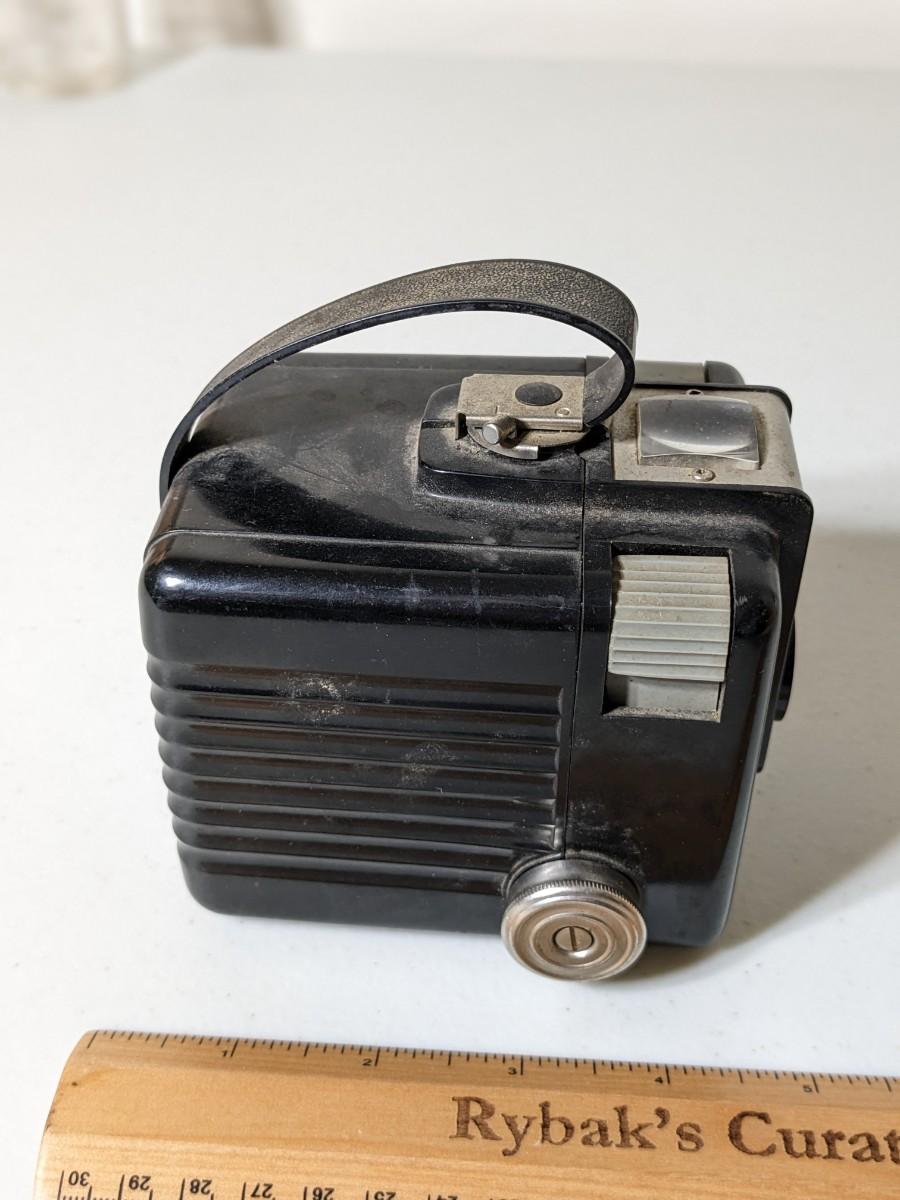This image showcases a vintage Brownie Hawkeye camera, viewed from the side against a completely white background. Dominantly black in color, the camera features a visibly worn black leather handle looped over the top. The handle appears slightly aged, indicative of its frequent use. The front of the camera includes a prominent latch, designed to open its back. A clear glass viewfinder with a gray trim is positioned at the top, with a side-mounted gray shutter button below it, accompanied by several other buttons on the top.

A notable metal component, a silver-colored circular dial, is located at the bottom right portion of the camera. The side of the camera showcases ridges, adding to its utilitarian design. Below the camera, a wooden ruler lies horizontally, providing context for the camera's size. The ruler is marked "RYBAX curate" and has measurements up to five centimeters visible. This ruler indicates that the camera is approximately four and a half inches in length. The image exudes a sense of nostalgia and highlights the detailed craftsmanship of the early photographic equipment.